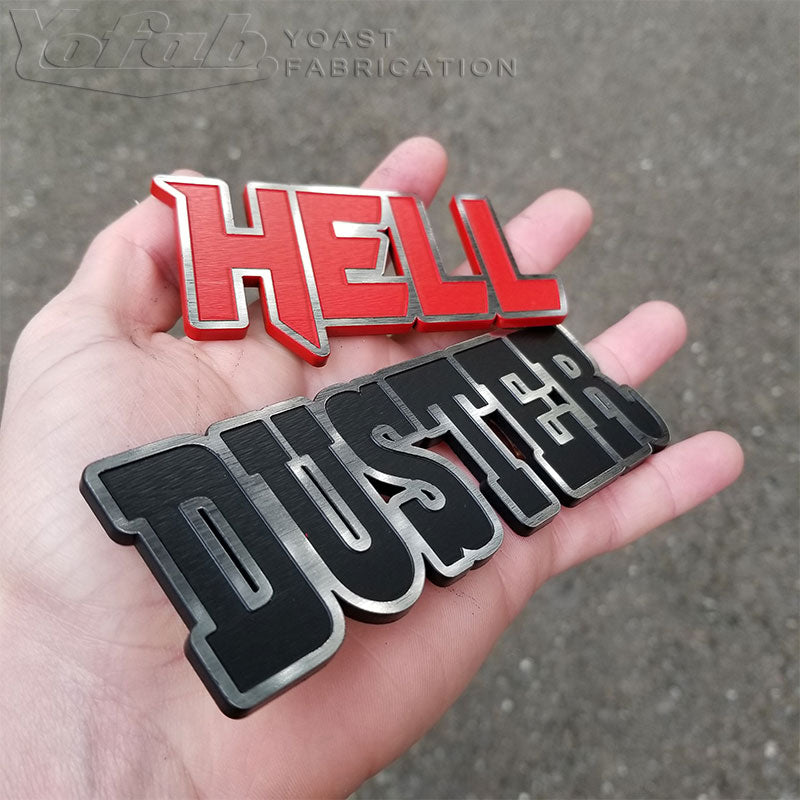This color photograph, taken outdoors, is a detailed close-up of a white hand extending from the lower left corner, holding two emblems or placards. The top emblem, inscribed with the word "HELL," features bold red letters with a silver outline, and the bottom emblem, labeled "DUSTER," has black letters outlined in silver. These emblems cover almost the entire palm of the person's hand. The background is blurred but suggests an outdoor setting, potentially a gravel or stony area that could be near an academy or similar stone structure. In the upper left corner of the image, a transparent overlay reads "YoFab Yoast Fabrication," indicating that this might be an advertisement for a company specializing in fabricating these types of metal pieces. There are no other significant details in the foreground or background.